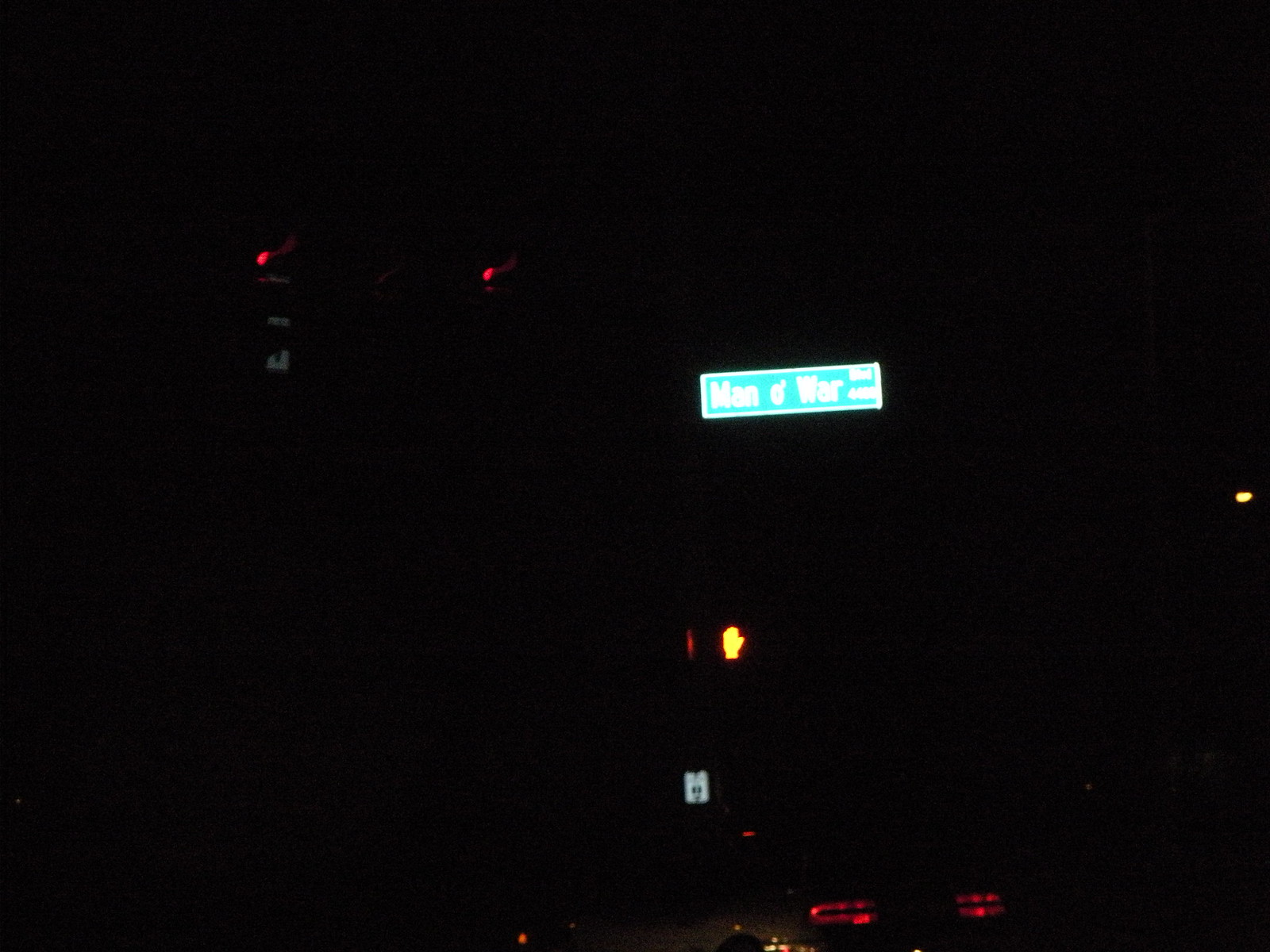In this captivating nocturnal scene, the darkness of the night envelops a quiet intersection, setting a somber mood. Prominently hanging overhead are two traffic lights, both glowing a deep red against their black casings, signaling caution to any approaching vehicles. The surrounding area is punctuated by the warm glow of a few scattered street lamps.

To the left, a green street sign with bold white lettering reads "Man of War Road," hinting at the location. Underneath this guiding marker, a pedestrian signal displays either a white or yellow hand, commanding attention and offering guidance to those on foot. Beneath this, another small white sign adds an additional layer of instruction for pedestrians.

To the right, the scene is accented by an array of car lights; a cluster of red lights glimmers in a semicircle, suggesting the presence of vehicles waiting at the signal. Additionally, the ambient light from distant street lamps gently illuminates various parts of the intersection, adding depth and texture to the night.